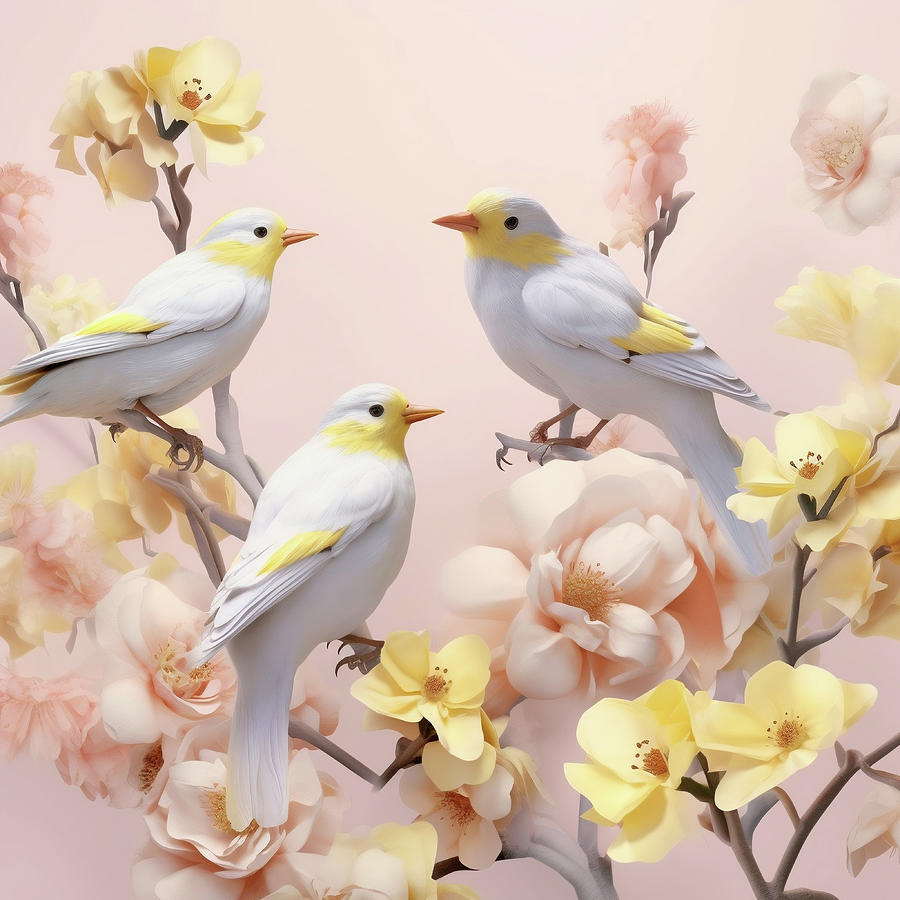This detailed painting captures a serene scene featuring three birds perched on delicate, flower-laden branches against a pale peachy pink background. The birds, primarily white with streaks of yellow on their heads, wings, and shoulders, sport bright orange beaks and small black eyes, offering a lifelike charm. Arranged thoughtfully, two birds face the right while one faces the left, creating a balanced composition. The branches, which meander gracefully from the upper left to the bottom and back up towards the upper right, are a mix of grayish-brown and green hues. They are adorned with an array of flowers, including small, thin light yellow blossoms and slightly bushier pale pink ones, reminiscent of dogwood flowers. The image, possibly square in shape and six inches on each side, presents a harmonious blend of nature's beauty in subtle yet captivating detail.